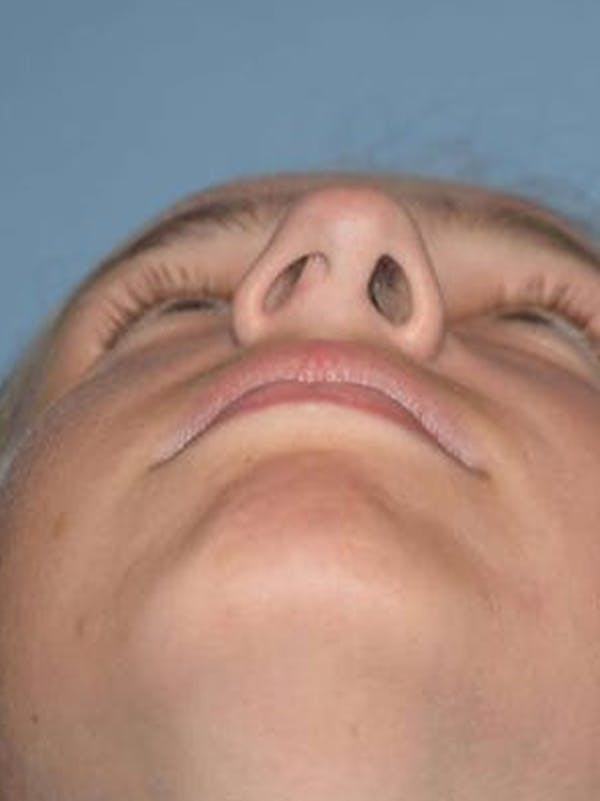In this unconventional image, the focus is on an upward-angled close-up of a person's face, taken from just below the chin, creating an almost exaggerated perspective. The image prominently displays the chin, slightly open lips, nostrils, and eyes looking upward. The face's features are vividly detailed; you can see the curves of the lips, the nostrils, even the fine hairs inside them, the eyebrows, and the long eyelashes. The background appears to be a bluish-gray color, adding a muted contrast to the tan, brown, and pink tones of the person’s face. Some stray hairs are visible at the top of the frame, though the rest of the hair and head are not apparent. The angle makes it seem like the person is taking a selfie or having their picture taken from a very low vantage point, possibly in a casual setting like their home.